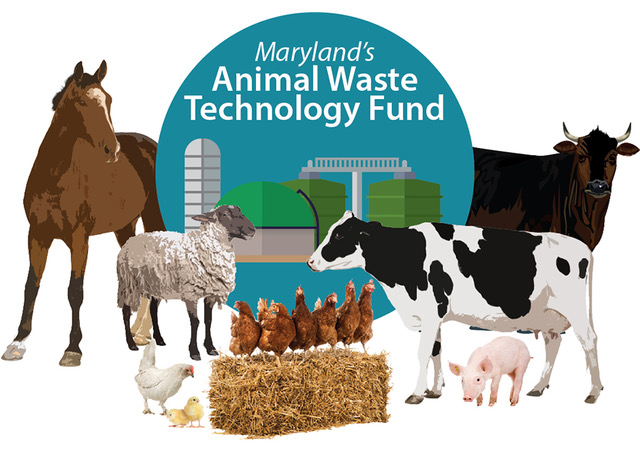The image features a circular blue emblem at its center with the white text "Maryland's Animal Waste Technology Fund." Inside this circle, there are graphics suggesting an industrial setting, including a couple of containment barrels. Surrounding the circle is an array of farm animals depicted in a stylized, almost photorealistic clipart manner. 

On the left side outside the circle, there is a brown horse with a distinctive white stripe on its head and white hooves. Next to the horse is a white chicken on the ground, accompanied by two yellow chicks. Below these, a row of six chickens, darker in color, stand atop a hay bale. To the right of the horse is a sheep. 

On the right side of the image, a piglet nestles under a dairy cow which faces left; this cow is primarily white with black spots. Above this cow is a large brown bull, facing forward with a steadfast gaze. Throughout the image, each animal is rendered with textured detail that blends lifelike elements with a graphically enhanced clipart style.